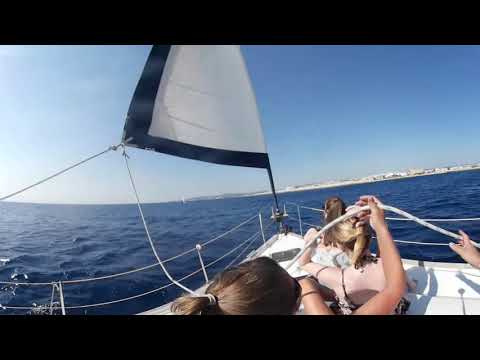In the photo, we see a small white recreational sailboat with an open top, carrying four people, including the photographer. The day is sunny with a completely clear sky, and the ocean stretches out around them. In the distance, land is visible, suggesting they might be heading there. The boat features a sail with a blue end, indicative of a gentle breeze helping their journey. Ropes are attached to the sail, which is fully extended. Three young white women in their early 20s to 30s, wearing swimsuits and some with sunglasses, are seated and facing forward, looking out at the water. A hand can be seen on the right, presumably belonging to the person taking the picture. A flag is spotted towards the top of the boat. Overall, the scene depicts friends enjoying a leisurely sail on a clear, beautiful day in the middle of the ocean. The colors in the image include shades of black, light blue, off-white, gray, brown, and yellow, with a black border at the top and bottom of the picture.